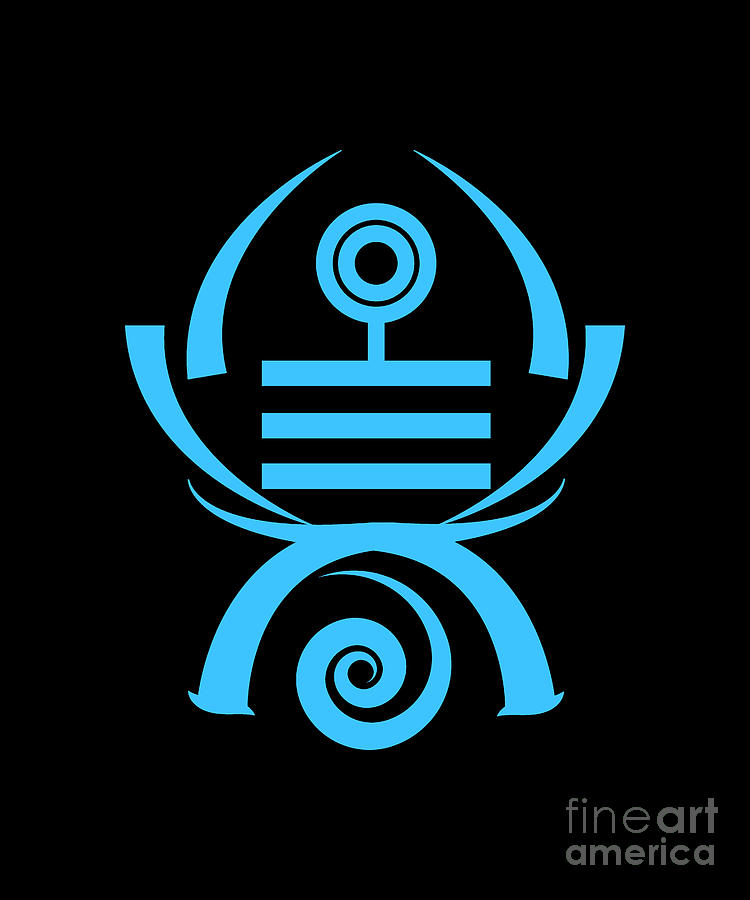This image appears to be an advertisement for Fine Art America, featuring a striking, tribal-inspired emblem centrally placed against a black background. The emblem is a vibrant, almost neon blue, which stands out starkly against the black. Central to the design are two curved lines that originate from a point at the top and gracefully extend downwards, flanking a circular motif. This circular motif consists of an outer blue circle encompassing a thin black ring, another blue circle, and a smaller black circle at the center. Below this, the motif extends down with a vertical line that connects to three evenly spaced horizontal lines.

Adding to the intricate design, there is an upside-down U-shape at the base, with a distinctive swirl pattern within it that starts from the top left, spirals down, and then loops towards the right. This swirl is encompassed by the two primary curved lines, which curl upwards from the base to nearly meet at the top.

The words "Fine Art America" are displayed in light gray at the bottom left corner of the image. The emblem's blend of geometric shapes and fluid lines lends it a dynamic and compelling visual appeal, evoking a sense of artistic sophistication.